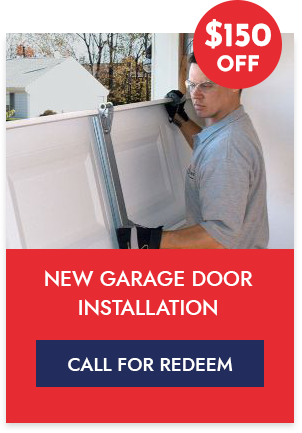A detailed caption for the image could be:

"This advertisement features a garage door installation service. The ad is divided into two main sections. The upper half showcases a photograph of a technician in the midst of installing a garage door. The technician is equipped with safety goggles and gloves, and is using a tool to maneuver the garage door onto its track, elevating it to eye level. In the background, a residential house and some trees are visible, adding context to the setting.

A prominent red circle with bold white text is partially overlaying the upper portion of the photo. The text within the circle reads '$1.50 OFF,' drawing immediate attention to the discount being offered.

The lower half of the ad features a solid red background with bold white text, clearly stating 'NEW GARAGE DOOR INSTALLATION.' At the very bottom, there's a large blue button extending across most of the width of the ad, with the text 'Call for Redeem' in white, urging potential customers to take action and redeem the discount."